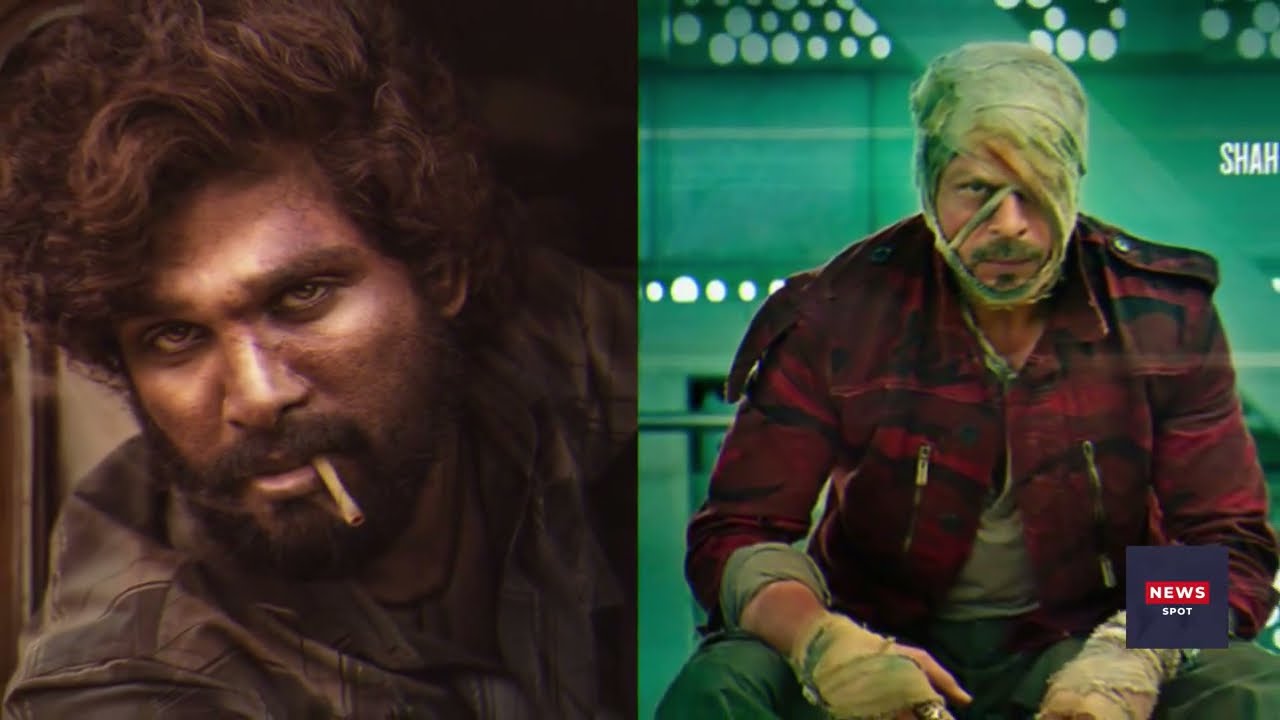The image comprises a side-by-side comparison of two distinct photographs of men, exuding a rough and gritty ambiance. 

On the left side, we have a man with curly, thick brown hair and a scruffy beard and mustache. Dirt smudges his skin, enhancing his rugged appearance. He wears a dark gray and black plaid shirt that’s visibly filthy, and a rolled-up cigarette dangles from his mouth. His intense gaze is directed straight at the camera.

On the right side, a younger man, also looking directly at the camera, has his face and head swathed in gauze, revealing only his left eye and part of his mustache and soul patch. Bloodstains mark the white gauze, indicating recent injuries. He dons a red and black camouflage jacket over a t-shirt, with his hands crudely bandaged. His disheveled attire and the presence of lights behind him suggest a stark, possibly urgent setting. The bandage extends across his nose, adding to his severely injured appearance, and his green pants complete the ensemble.

In the lower right-hand corner of the image, the word "news spot" is visible, hinting at a potential context or source. The men’s intense, menacing expressions, combined with their battered and gritty appearances, suggest a scene of hardship or confrontation. The color palette features black, brown, tan, white, gray, green, red, and maroon, reinforcing the image's stark and dramatic tone.